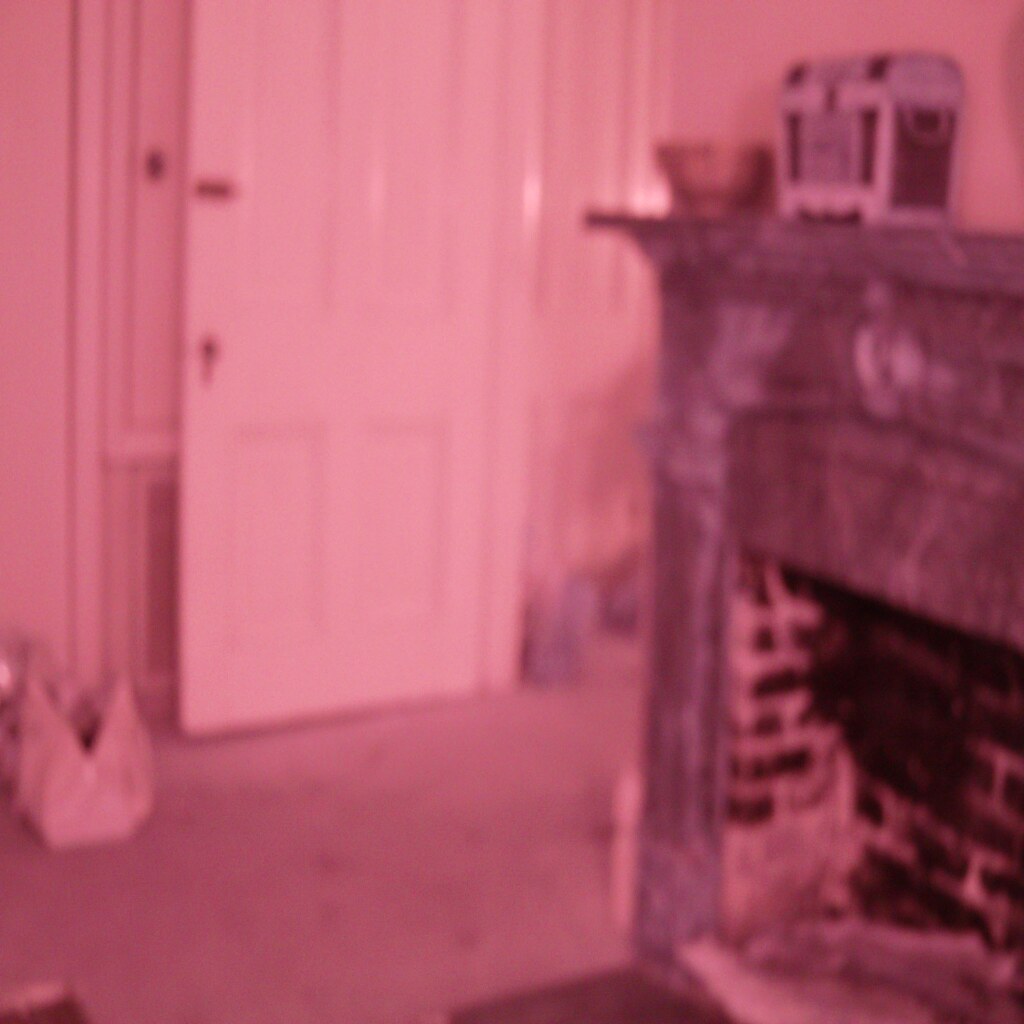The image is a blurry photograph with a sepia or reddish tint. On the left side, a closed, presumably white, door is visible. Adjacent to the door on the right, a brick fireplace dominates the scene. The fireplace is empty, with bricks lining the interior where a fire would typically burn. Atop the mantel, a small treasure chest sits, flanked by a bowl on its left side. The overall setting gives off a historical or antique ambiance.